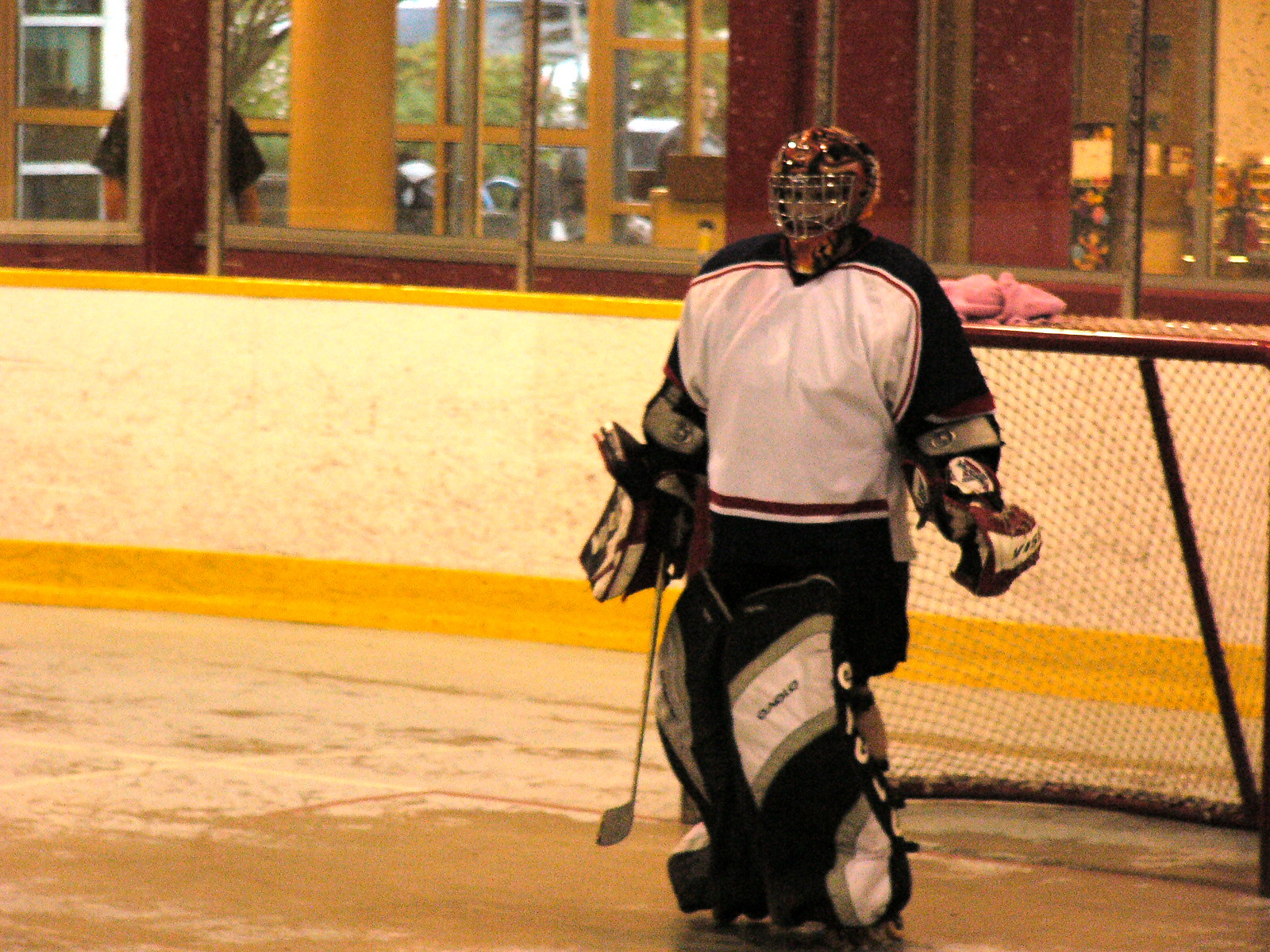The photograph captures a detailed scene from a roller hockey game taking place in a moderately-sized indoor rink, which appears somewhat worn with areas where the paint has faded, revealing a brownish surface underneath. At the center of the image stands the focal point, a goaltender poised in front of the goalie net. The goaltender is dressed in a white and black jersey accented with red lines, sporting an orange and black helmet with a full face mask, and holding a stick by his side. Though the arena resembles a typical ice hockey rink, closer inspection of the player's roller skates confirms the absence of ice, identifying it as a roller hockey setting. The surrounding environment includes the standard rink boards topped with protective plexiglass. Beyond the rink, there are indistinct rooms and some figures moving about. The overall atmosphere suggests an amateur or recreational setting rather than a professional one, underlined by the rink’s modest size and lack of spectator seating.